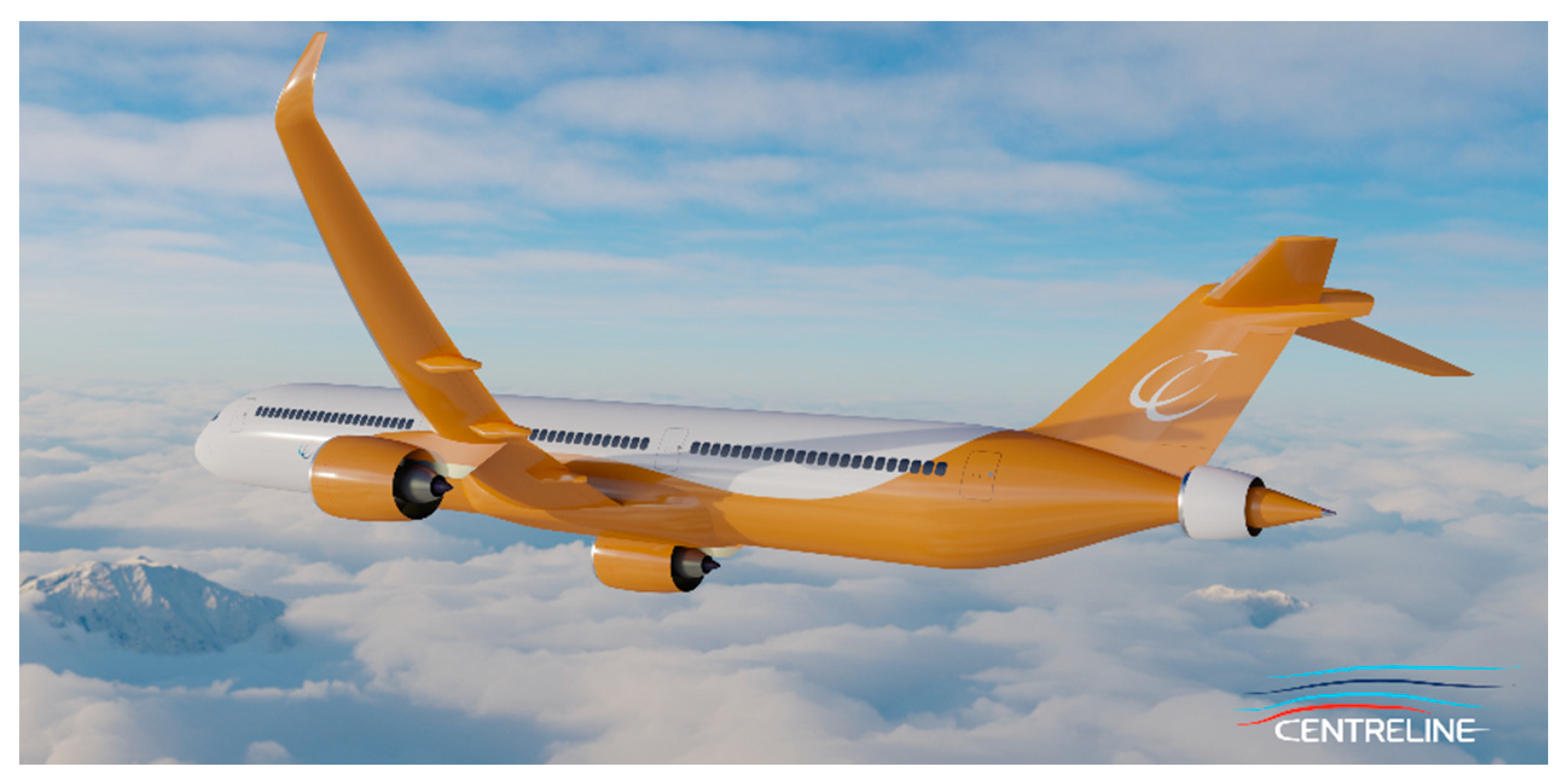This is an old advertisement, likely from the 50s or 60s, featuring an illustration or a colorized picture of a concept passenger airplane named "Centerline." The airplane is depicted as an enormous, elongated aircraft with three large compartments. It is colored in a vibrant popsicle orange and white, soaring above a sea of puffy, beautiful clouds under a light blue sky. Some clouds have broken open to reveal snow-capped mountaintops below. The scene suggests either a sunrise or sunset due to the sun's reflection on the clouds. The airplane appears to be in the process of turning to the right, with its left wing angled upward. The right wing has two white half circles. The tail of the airplane features a distinctive bee stinger shape with a white ring around it. On the bottom right corner of the image, the text "CENTERLINE" is visible along with a company logo that includes blue and red lines above the word. The illustration captures the aircraft from a viewpoint slightly below, enhancing its grandeur and the sensation of flight above the clouds.